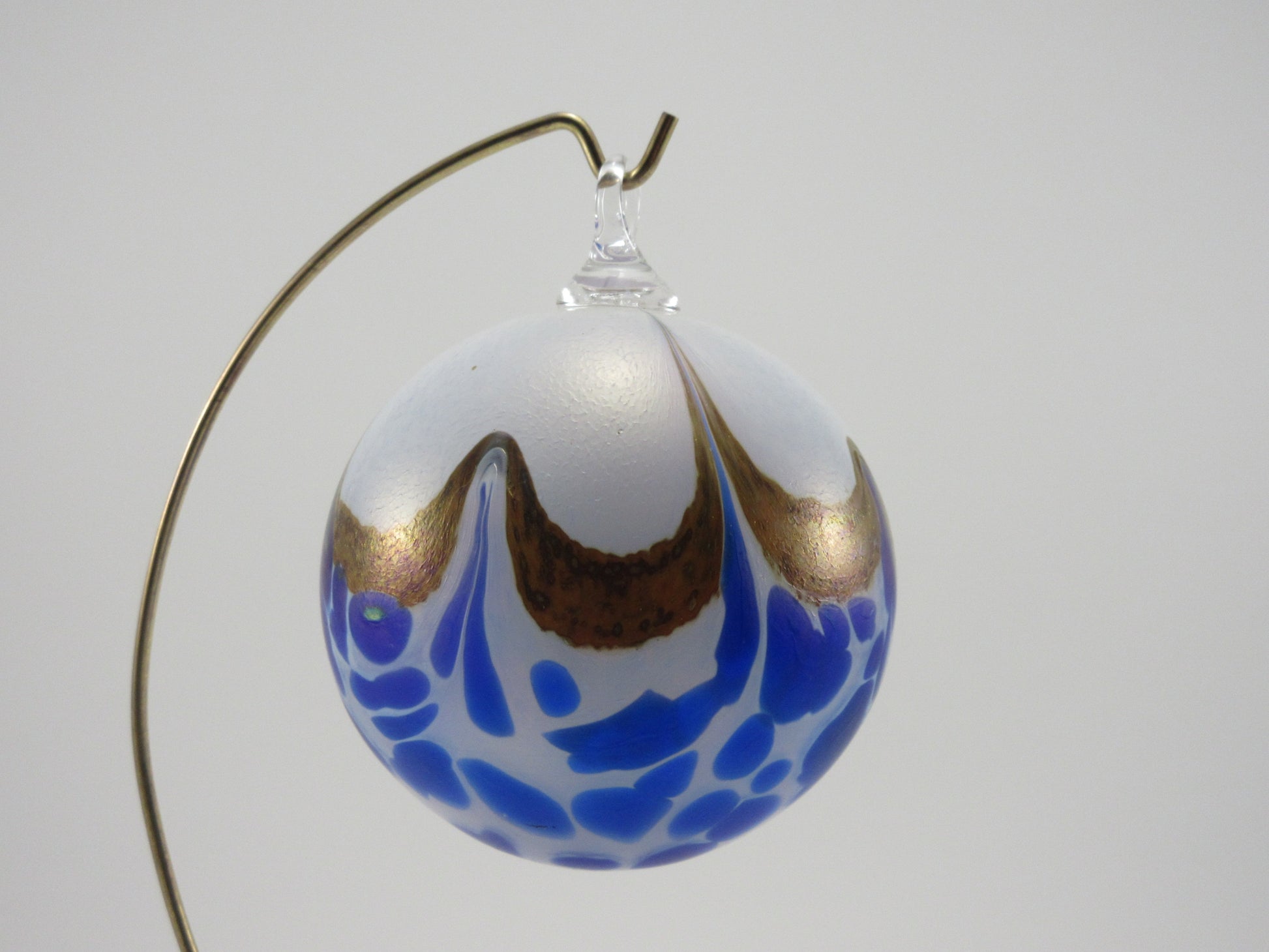The image showcases a close-up of a hand-blown Christmas ornament against a light gray, almost white background. The ornament hangs from a golden metallic wire stand that originates from the lower left corner, curving upwards to form a hook at the top. Attached to this hook is the ornament, featuring a clear, circular attachment at its top for hanging. 

The ornament itself is a perfect sphere with a distinctive design. The top portion is predominantly white, resembling dripping paint that transitions seamlessly into a gold or bronze section, which further trickles down into the ornament. The bottom half of the sphere is adorned with blue circular shapes and lines, giving the appearance of blotched or dripped glass. Additionally, there are repeating U-shaped golden scallops encircling the midsection, adding an extra layer of intricate detailing. The overall aesthetic is that of a delicate and elegantly adorned Christmas bulb, free from any external text or figures.